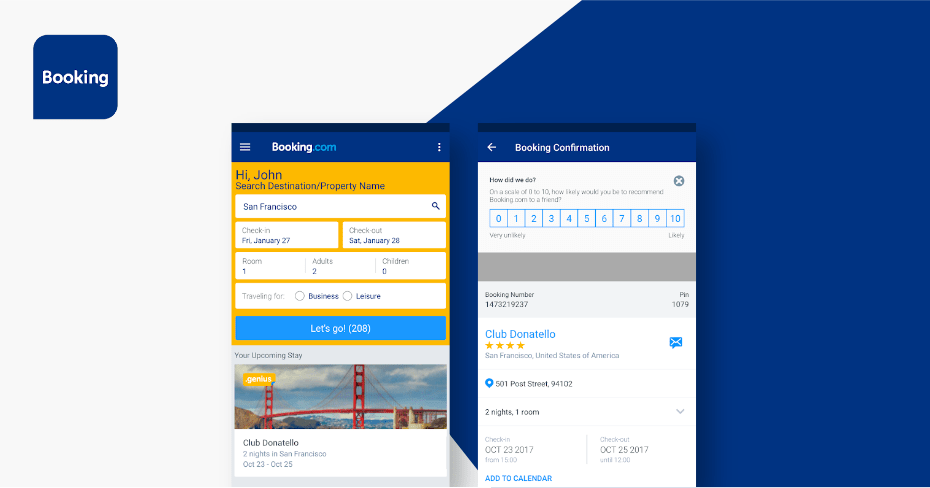This image is a screenshot taken from the Booking.com app, featuring two distinct screens within the app interface. The first screen is a welcoming page addressed to a user named John. It includes a search bar with the placeholder text, "Search Destination or Property Name," allowing users to enter their desired city, travel dates, and the number of guests. A prominent "Let's Go" button, in a light blue color, encourages users to proceed with their search. Additionally, there is an image resembling the Golden Gate Bridge enhancing the visual appeal of this screen. 

The second screenshot displays a feedback or survey prompt, asking users how their experience has been with the app. Below this prompt, there is an itinerary overview for a trip scheduled from October 23rd to October 25th. In the top left corner of both screenshots, the Booking.com logo is visible—a dark blue square featuring the text "Booking" in white.

The overall layout of the app is divided into a white and blue color scheme, with the left side predominantly white and the right side blue, providing a clean and organized user interface.